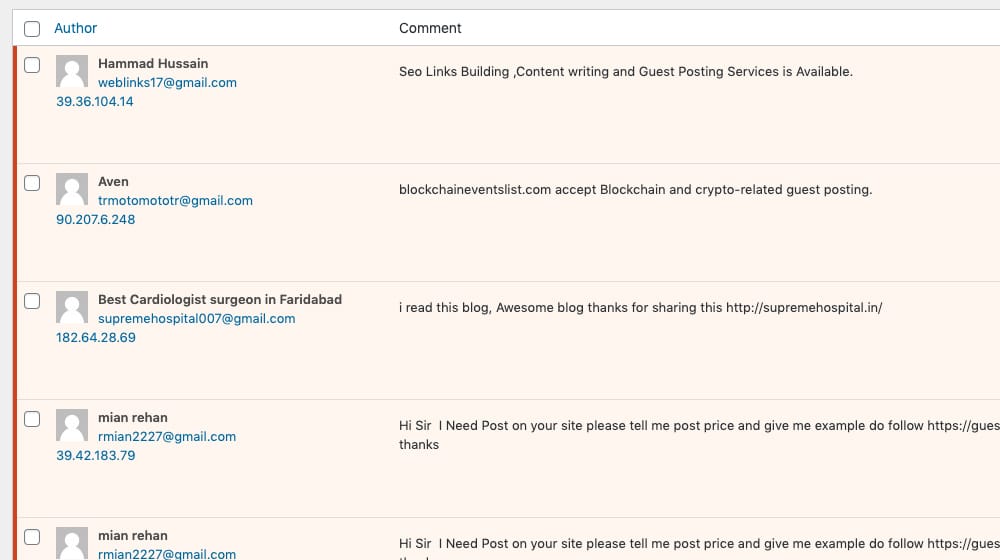The image displays a beige page entitled "Author" in blue text at the top left corner, while "Comment" is written in black text on the right. The page contains multiple comments from various individuals, totaling five comments in all.

1. **Hamad Hussain**:
   - **Email Address**: weblinks17@gmail.com
   - **Comment**: "SEO links building, content writing, and guest posting services are available."
   - **Additional Element**: Some kind of code is shown in blue beneath the comment.

2. **R Even**:
   - **Website**: blockchaineventslist.com
   - **Comment**: "Accepts blockchain and crypto-related guest posting."

3. **Best Cardiologist Surgeon in Faridabad**:
   - **Comment**: "I read this blog. Awesome blog, thanks for sharing this!" 
   - **Additional Element**: Includes a hyperlink.

4. **Mian Rehan (First Comment)**:
   - **Comment**: "Hi sir, I need posts on your site. Please tell me the post price and give me examples. Do follow."
   - **Additional Element**: Includes a hyperlink.

5. **Mian Rehan (Second Comment)**:
   - **Comment**: Repeats the same comment as his first one, i.e., "Hi sir, I need posts on your site. Please tell me the post price and give me examples. Do follow."

Each comment includes the name of the commenter located to the left, with additional details such as email addresses, service offers, website links, and requests for guest posting opportunities.